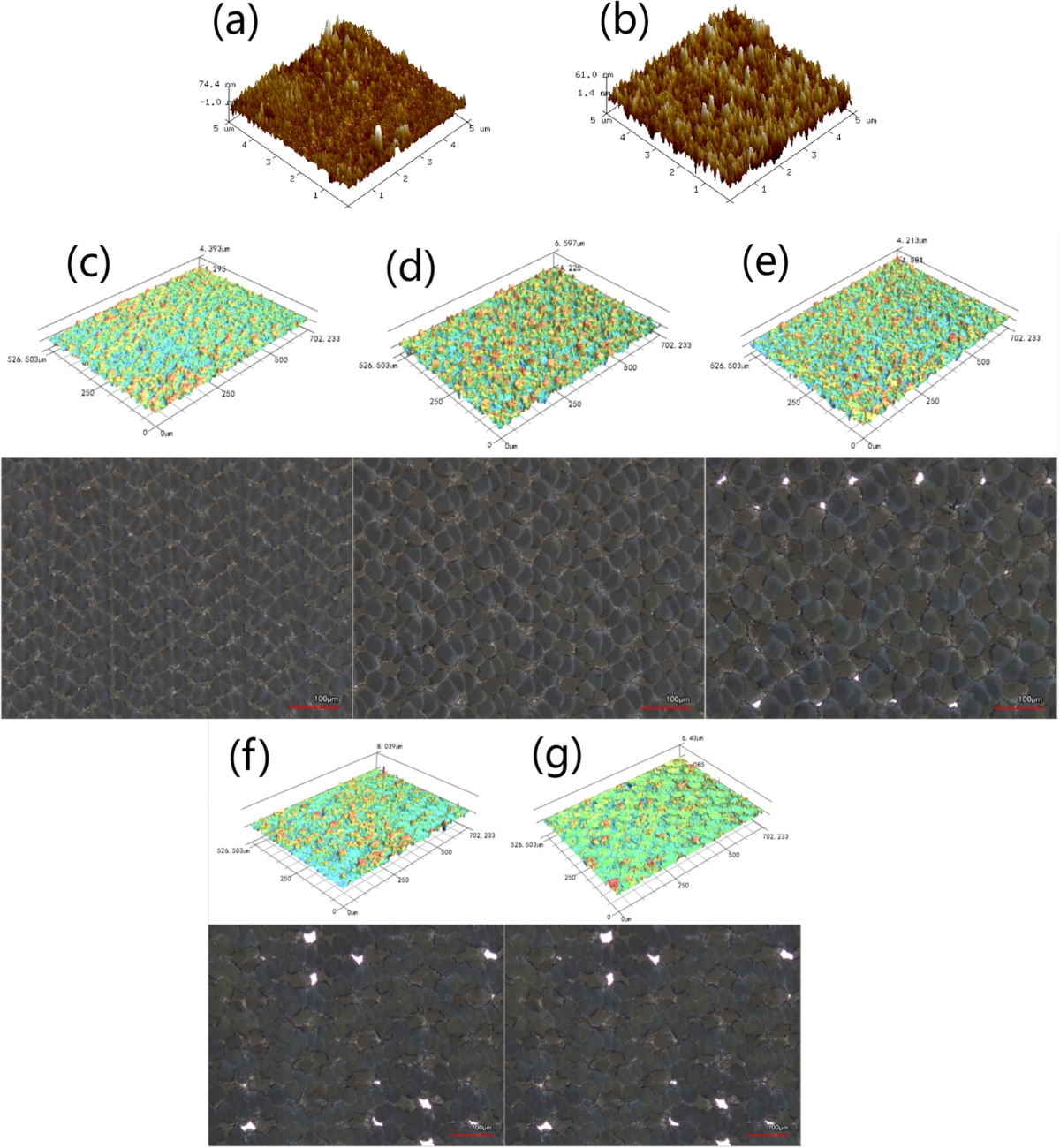The image is a detailed diagram that showcases a series of charts, resembling topographical maps with various renderings. At the top, there are two square charts labeled A and B, featuring what appear to be tree covers in fall colors, with A showing denser foliage and B having a more yellowish tint. Beneath these, there are three rectangular diagrams labeled C, D, and E, predominantly displaying multicolored, mainly blue and green textures. Below them are three zoomed-in gray images resembling scales or bubbles, which exhibit intricate patterns of white light within the gray. Further down, there are two additional rectangular diagrams labeled F and G that continue the blue and green color scheme, with two more gray, scale-like images situated beneath them. Each section of the diagram is meticulously labeled from A to G, indicating different sets of data or textures in a structured layout.